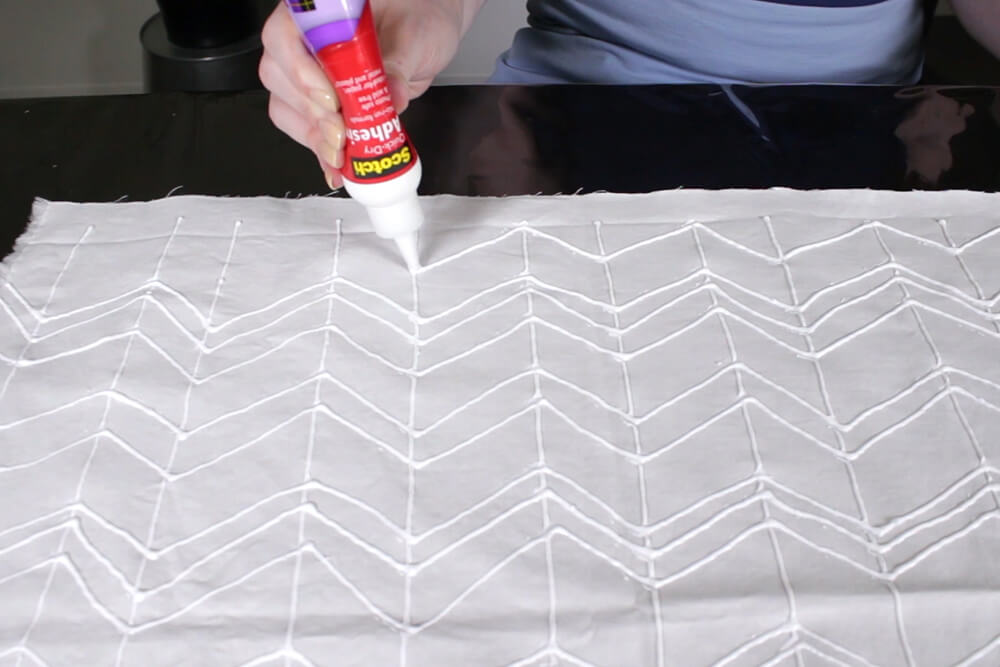In this instructional photo, commonly found on platforms like YouTube, a person with fair skin is seated at a shiny black table, applying adhesive to a piece of light gray fabric. The individual, dressed in a blue shirt, grips a scotch adhesive bottle in their right hand. The bottle, which is upside down, features a red body with white and yellow lettering, a purplish bottom, and a white cap, clearly labeled "scotch adhesive." The adhesive being dispensed is white, resembling Elmer's glue.

The person is creating a detailed pattern on the fabric, with lines forming a chevron design interspersed with perpendicular lines at various intervals. The bottom three-quarters of the image prominently displays the fabric and pattern, while in the upper portion, the person's hand enters from the top left corner of the frame. The background reveals a room interior, with a visible wall and top molding of a baseboard, along with two stacked cylindrical objects that resemble barrels or buckets. Reflections from the black table surface are also visible. This detailed instructional image captures the meticulous process of adhesive application on fabric.